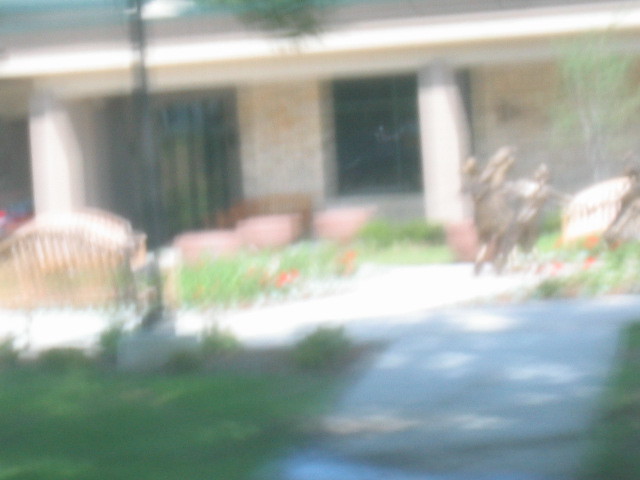In this extremely blurry photograph taken on a sunny day, we can discern an outdoor setting with a sidewalk flanked by patches of grass on both the left and right sides. In the upper part of the image, there is a structure that is likely a building or house, featuring pillars or columns that might be supporting a roof or porch. To the right of this area, near what could be the front door, there are a couple of indistinct figures whose actions are indeterminable due to the blurriness. The image contains no text.